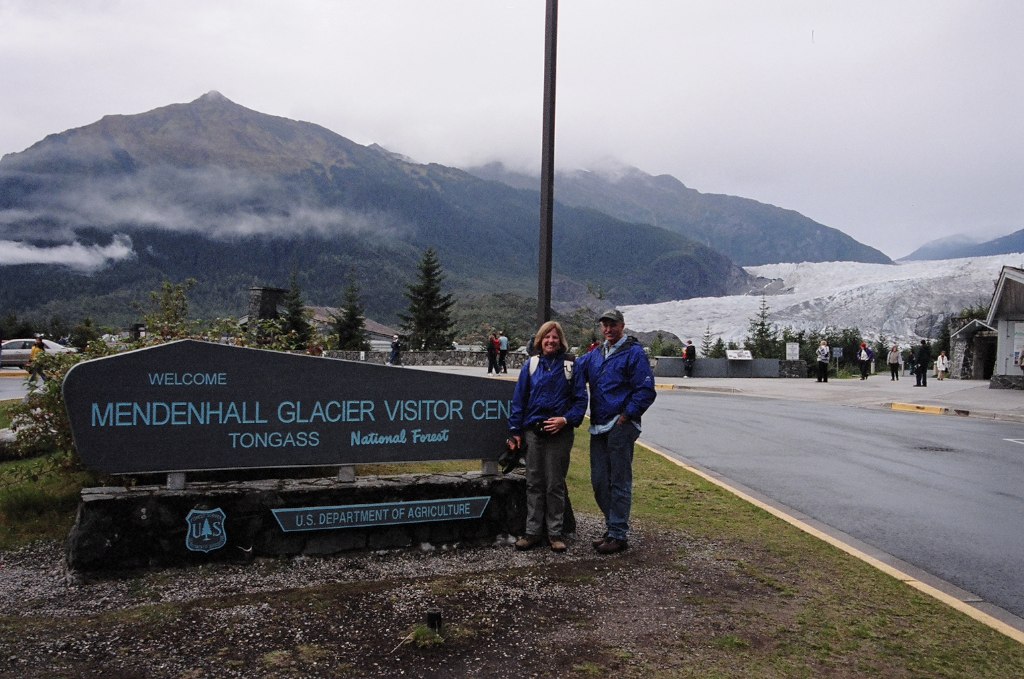In this photo, two individuals—a man and a woman, both dressed in matching blue windbreaker jackets and gray pants—stand with their arms around each other in front of a sign that reads, "Welcome Mendenhall Glacier Visitor Center, Tongass National Forest, U.S. Department of Agriculture." The woman, sporting shoulder-length blonde hair and a backpack with white straps, is smiling warmly, while the man, smiling as well, wears a gray ball cap. They are the main focus of the image. Behind them, fog drapes over majestic mountains that appear almost smoky, creating a mysterious and ethereal atmosphere. To the right of the couple, there's a roadway with people walking on a sidewalk, and a small building with a roof is visible. Snow patches and grassy areas lie at the feet of the mountains, adding to the landscape's contrast. Further in the background, the expansive Mendenhall Glacier can be glimpsed, enhancing the grandeur of the scene.